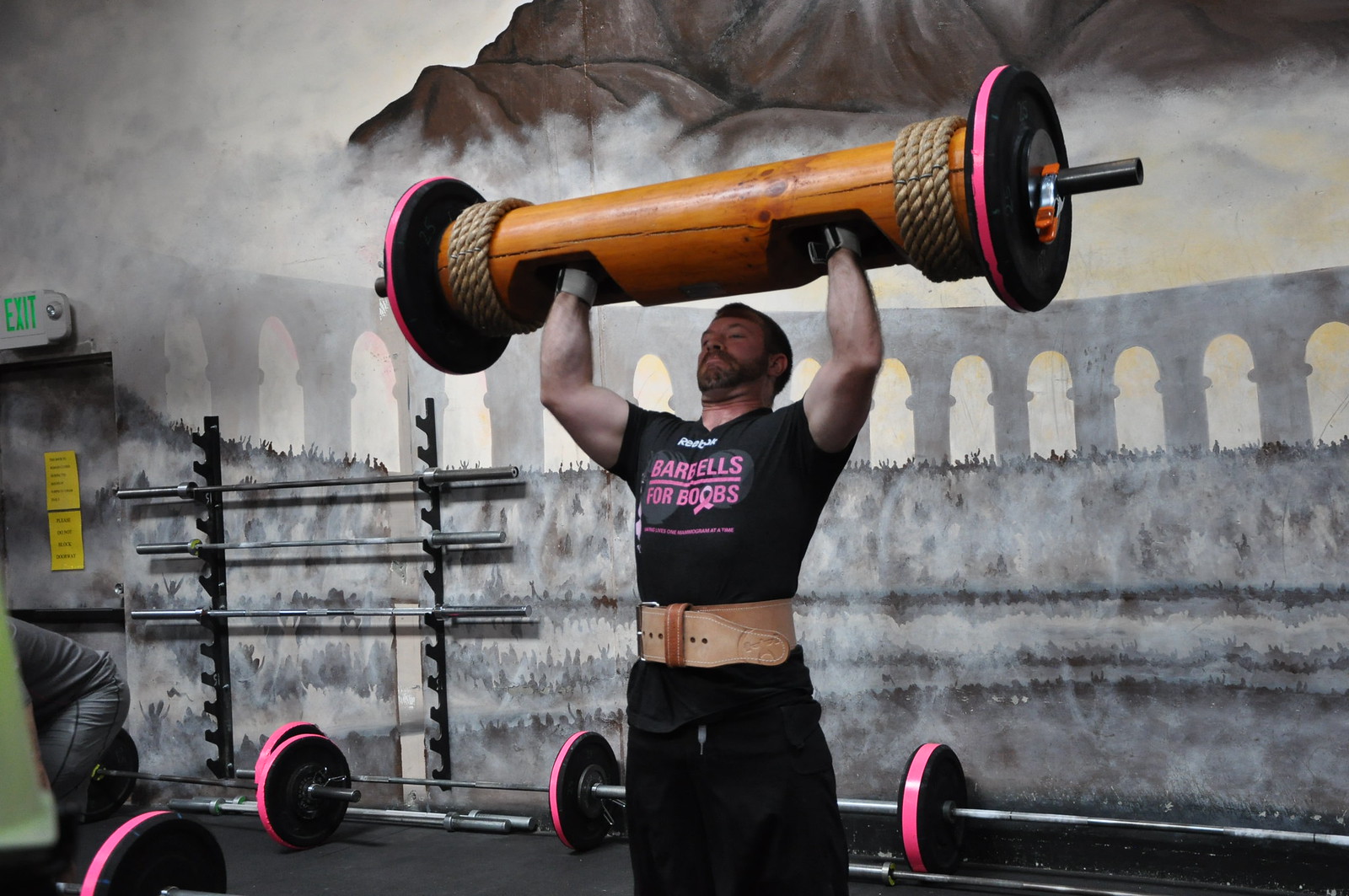The image, taken in color, showcases a spacious CrossFit gym with high ceilings and an airy interior. Dominating the scene is a strong-looking man, likely in his 30s or 40s, with substantial biceps prominently displayed as he lifts a unique barbell overhead. This barbell, made to resemble a large pole with wood and rope elements, features weights on each end. These weights are black rimmed with pink stripes and are detailed with handholds and twists of rope. The man, wearing a black t-shirt emblazoned with "Barbells for Boobs" and a leather weightlifting belt cinched tightly around his waist, stands in front of a mural. The mural depicts gray Roman viaduct arches set against brown mountains and clouds, adding a dramatic backdrop to the scene. Various barbells and dumbbells are scattered across the floor, and there's a rack storing more lifting bars in the far left corner. A yellow notice is posted on a door integrated into the mural, with an exit sign illuminated in green above it. In the distant corner, another person is visible, contributing to the dynamic atmosphere of this expansive and uniquely decorated gym.